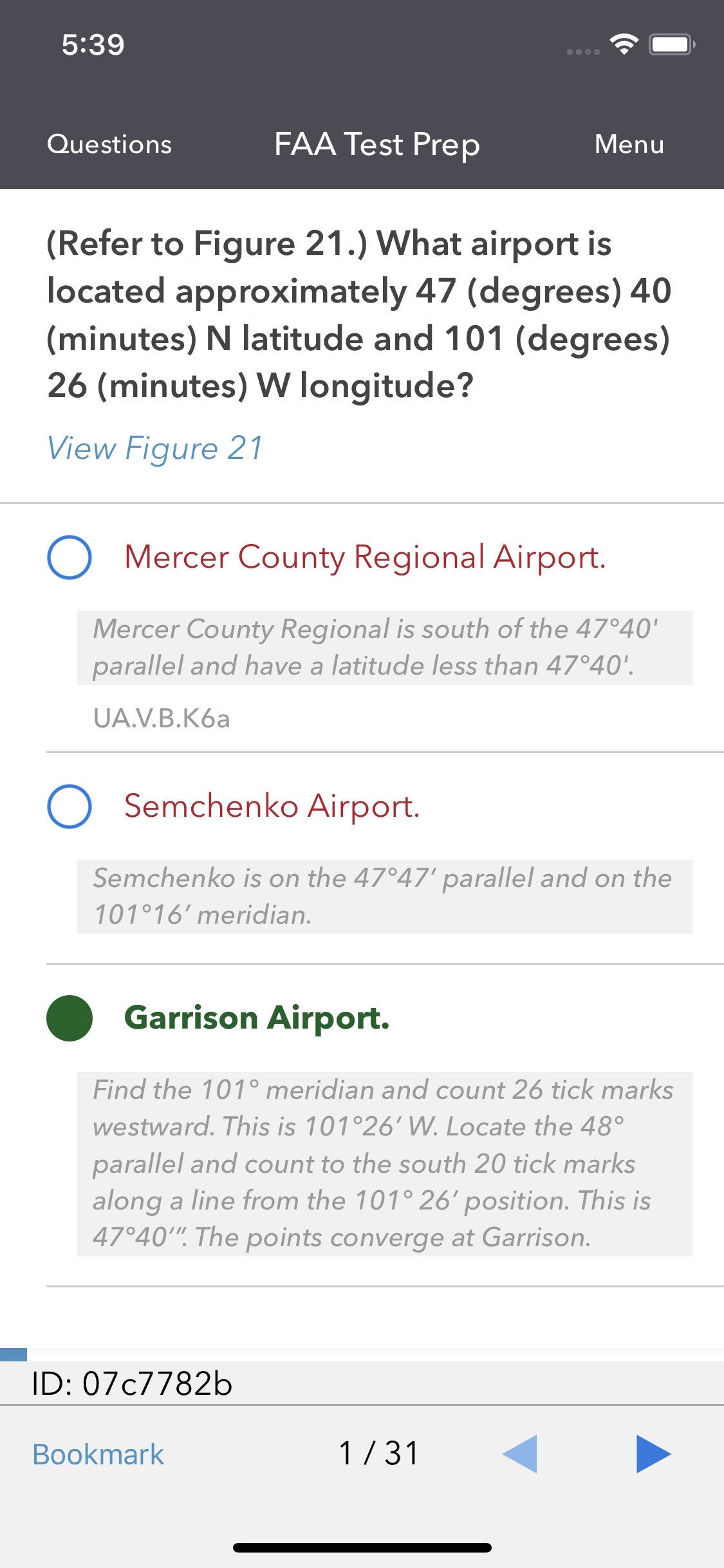The image displays a test preparation screen for the FAA, viewed on a mobile phone. In the top right corner, there are four dots representing a menu, positioned next to the Wi-Fi signal and a full battery icon. The header reads "FAA Test Prep."

Directly below the header, there is a section labeled "Figure 21" in brackets, which is followed by the question: "What airport is located approximately 47 degrees 40 minutes north latitude and 101 degrees 26 minutes west longitude? View Figure 21." Beneath the question are three radio button options:

1. Berkshire County Regional Airport (displayed in red),
2. Simchenko Airport,
3. Garrison Airport (selected in green).

A detailed explanation is provided under the selected answer, Garrison Airport, highlighted in green. The description instructs to find the 101-degree meridian and count 26 tick marks westward to 101 degrees 26 minutes west latitude. Next, locate the 47-degree parallel and count 40 tick marks south along the line from the 101 degrees 26 minutes west position, converging at Garrison Airport.

At the bottom of the screen, there is an identifier: "ID 07c7782b," a gray line, and the text "bookmark, one of 31," along with navigation buttons for "back."